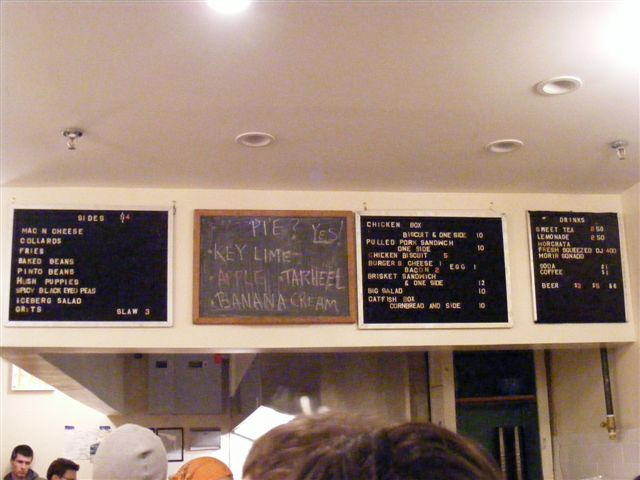The photograph captures the menu area of a cozy restaurant café, dominated by four chalkboards meticulously hung along a lower section of the ceiling that curves around the counter. The top part of the image prominently features these menu boards along with the ceiling and the tops of patrons' heads. In the background, a tall gentleman stands, possibly due to either his height or his position in the room.

The room is brightly lit, primarily from overhead lights, giving the entire space a vivid ambiance. The illumination blends with the white walls, casting a peculiar yet warm pinkish-yellow hue throughout the café. 

Each menu board details different categories of offerings, with one board specifically listing the sides available: macaroni and cheese, collard greens, fries, baked beans, hushpuppies, spicy black-eyed peas, iceberg lettuce, grits, and slaw. The prices for these sides range from three to four dollars.

Another chalkboard proudly advertises pies with charming handwritten notes, listing flavors such as key lime, apple, banana cream, and "tar heel." The main menu features heartier items including a “Chicken Box” (which comes with a biscuit and one side), pulled pork sandwiches, chicken biscuits, burgers and cheese with optional add-ons like bacon or an egg for an additional cost. More selections include a brisket sandwich with one side, a large salad, catfish, and cornbread.

The drinks menu showcases a variety of beverages – sweet tea, lemonade, horchata, fresh-squeezed orange juice, soda, coffee, and beer. 

Amidst the comforting, bustling environment of the café, the detailed menus and warm, lit atmosphere create an inviting space for patrons.